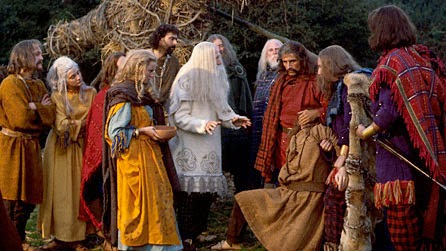This color photograph depicts a medieval scene where a group of about ten individuals, dressed in period-appropriate attire, witness a tense interaction. Central to this scene is a man with very long white hair, clad in a white and gray tunic, who appears to be attempting to mediate or intervene. Beside him, to his right, is a distressed man in a brown tunic, kneeling on the ground, possibly being restrained by another man in a red tunic who holds his hand over the kneeling man's mouth. The onlookers, comprising both men and women, are mostly dressed in shawls and vintage clothing, with the men sporting long hair and varied facial hair, ranging from white to brown. To the left, a large tree trunk covered in vines stands in the background, with a dense growth of green trees beyond it. The group seems deeply engrossed in the situation, with the women peering over the shoulders of the men to get a better view. The outdoor setting and detailed costumes lend a palpable medieval atmosphere to the scene.